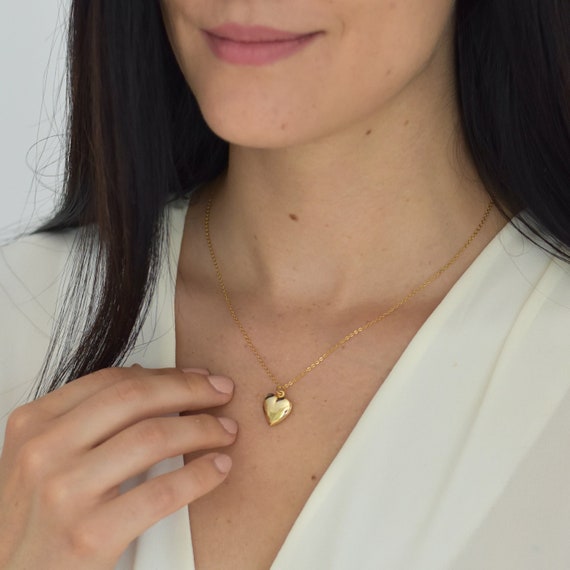The image depicts a close-cropped, color photograph of a Caucasian woman primarily highlighting a gold heart-shaped locket around her neck. The photo is centered on the area from just below her nose to a bit above her chest, focusing particularly on the locket. The woman has brown hair with darker tints and is wearing a sheer white blouse, through which her skin is slightly visible. Her hand, adorned with nude nail polish, rests near the locket, suggesting a posed stance for the photo. Her lips are curved into a slight, smirking smile. The locket, which appears polished and brand-new, hangs from a delicate gold chain. The photograph's plain white background further emphasizes the central subject of the locket.